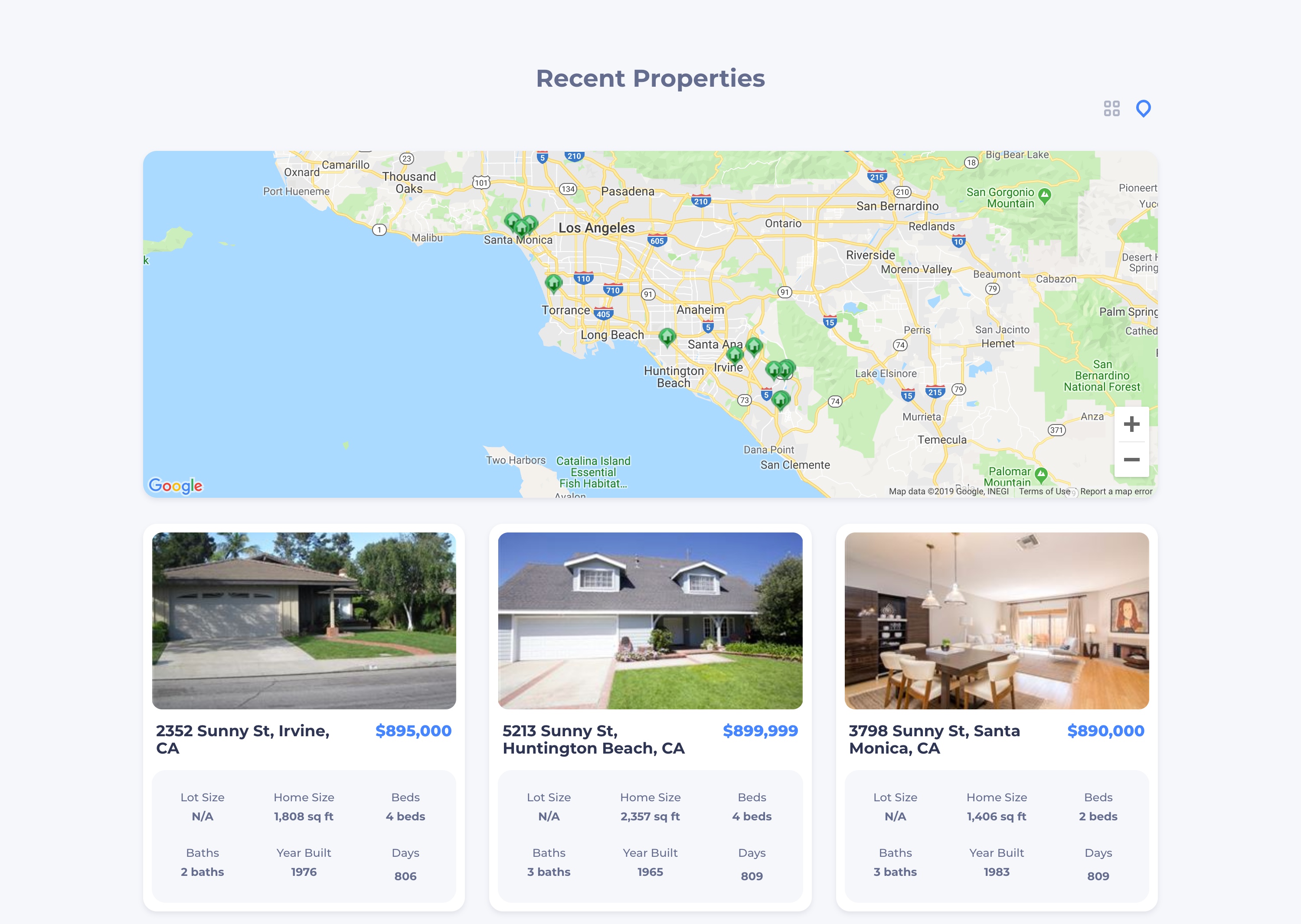The image displays a detailed map of the Los Angeles area, highlighting numerous potential houses for sale. The marked locations span a broad region, from Santa Monica down to Santa Ana and even Huntington Beach. The map, which uses Google Maps interface and allows for zooming in and out, serves as a comprehensive visual guide to the properties available. 

Beneath the map, there are photographs of specific properties accompanied by some essential details. The first property is located at 2352 Sunny Street, Irvine, California, and is listed at $895,000, with the price shown in blue on the right-hand side. Next is the property at 5213 Sunny Street, Huntington Beach, California, which appears to be slightly pricier at $899,999. Finally, there is the property at 3798 Sunny Street, Santa Monica, California, priced at $890,000. Each property photo also includes images of the interiors, giving a glimpse into the home’s design.

Beneath these photographs, further details about the homes are provided, such as their sizes, the number of bathrooms, and the year they were built, enhancing the overall understanding of each property’s value and characteristics.